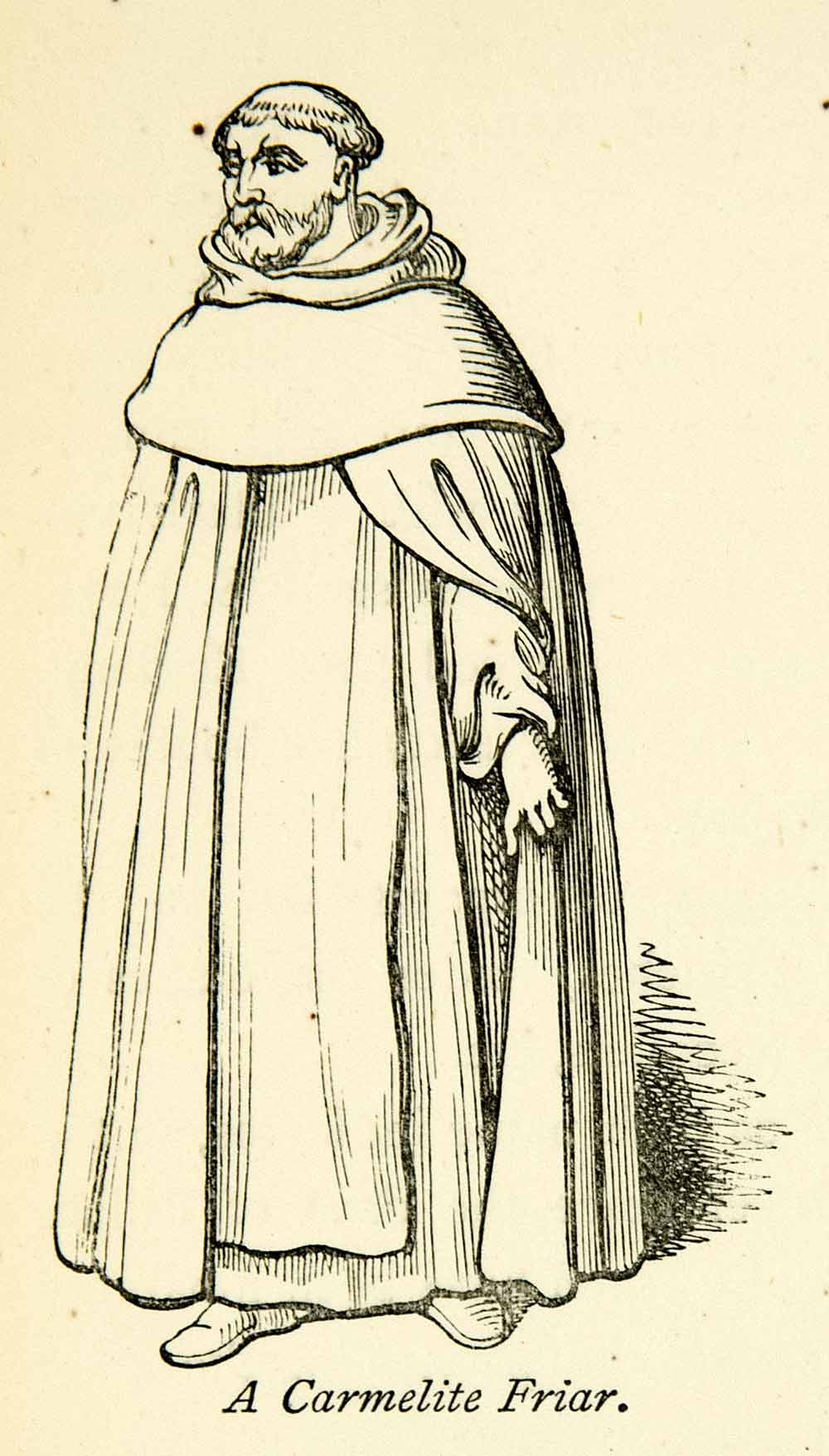This antique black and white illustration is rendered on a yellowed background, emphasizing its age and historical context. The focal point of the image is a man, depicted in profile, facing towards the left. His hair is styled in the traditional tonsure associated with monks, featuring a shaved crown and a ring of hair encircling it. His expression is marked by a frown, and his facial hair includes a full beard and mustache.

Draped around his form is a flowing, white robe, indicative of his religious vocation. The robe’s hem is lifted just enough to reveal his footwear. A cowl rests down over the back of his neck. The man's left hand is visible and relaxed at his side, while his right hand remains out of sight within the composition. Adding depth to the illustration, a scribbled marking behind the figure represents a shadow.

Inscribed at the bottom of the illustration are the words, "A Carmelite Friar," providing both a description of the figure and a clue to his identity. The meticulous spelling out of "Carmelite Friar" underscores the importance of accuracy in the captioning of this historical image.